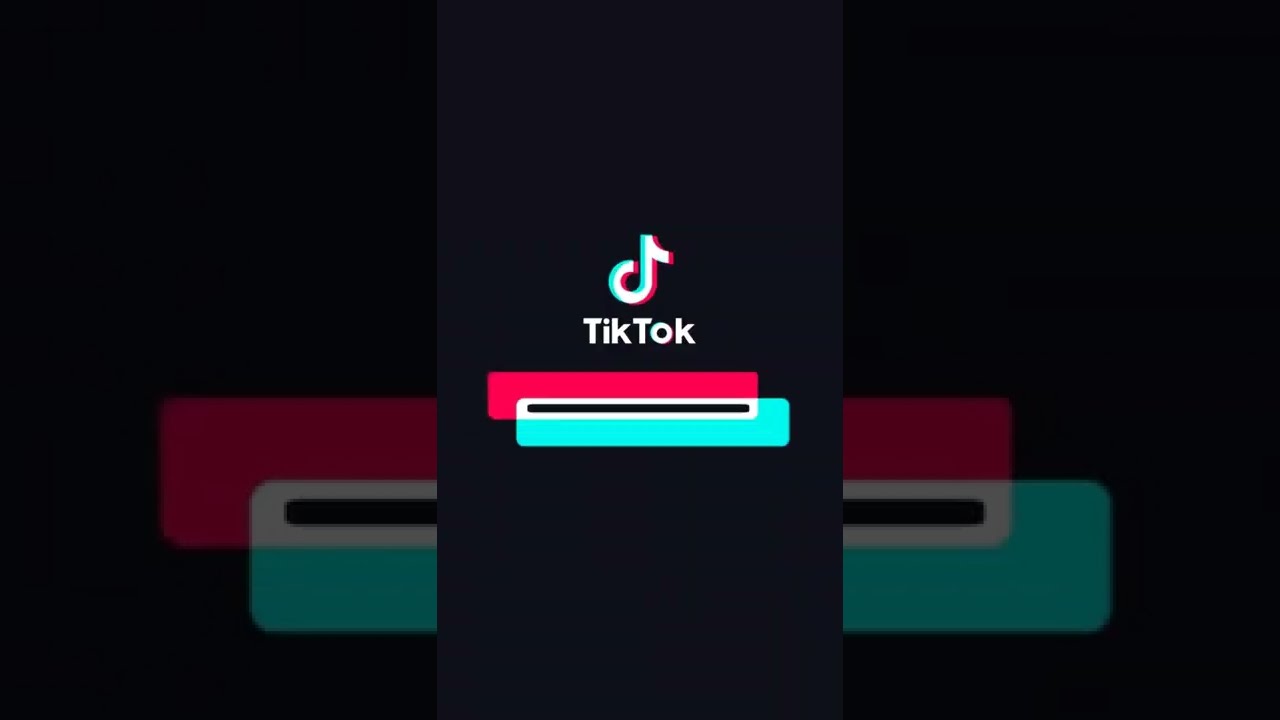This image, a vertical screenshot of a video, showcases the TikTok logo prominently in the center against a black background. The central section features the main TikTok logo, which includes the iconic music note symbol above the text "TikTok" in white letters. The logo is bordered with cyan on the left and magenta on the right. Below the logo is a red (magenta) bar and a blue (cyan) bar that overlap slightly, creating a thin, black rectangle with a white outline where they intersect. This overlapping section is typically where TikTok animates the username of the video's creator. On either side of the central image, the smaller sections of the red (magenta) and blue (cyan) bars are magnified, providing a closer look at these elements. The entire image is somewhat pixelated, indicating it is a low-quality screenshot.